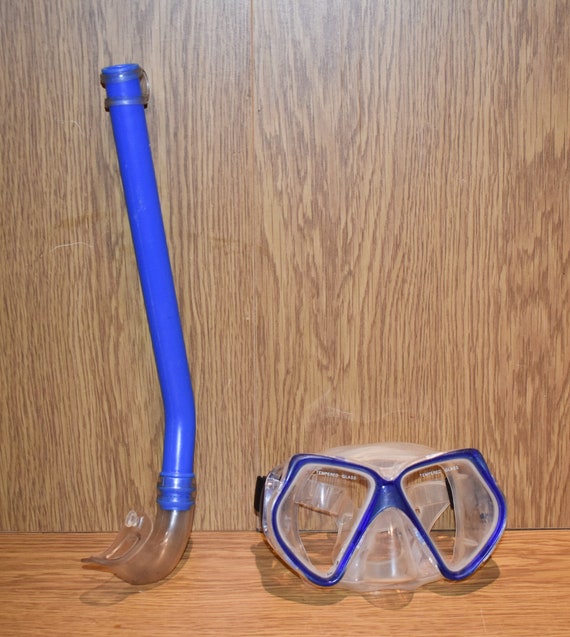The image showcases a detailed close-up of snorkeling equipment, carefully arranged on a wooden table with wood paneling in the background. On the right side of the image is a pair of snorkeling goggles. These goggles feature a clear plastic housing with a substantial blue frame encircling the lenses, which resembles the shape of glasses. The nose bridge of the goggles is also made of clear plastic. To the left of the goggles is a snorkel. The snorkel has a clear, opaque mouthpiece connected to a bright blue tube. The equipment appears tidy and clean, resting side by side in front of the grained brown wood backdrop, creating a harmonious and organized display.